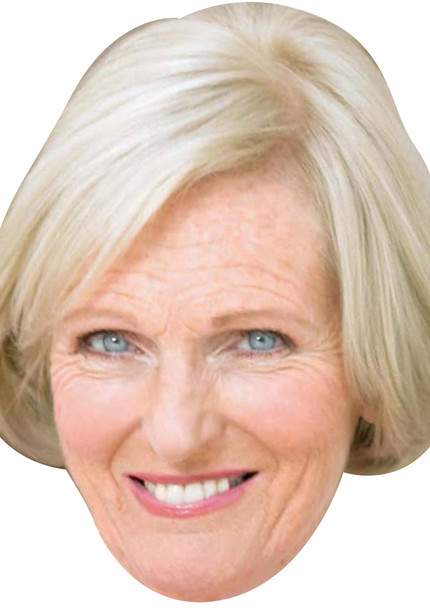The image features a close-up portrait of an elderly woman, prominently filling the entire frame against a plain white background. Her head is depicted from just below the chin upwards, excluding her neck. The photograph captures her light platinum-blonde hair, which is straight and parted to her left, sweeping across the right side of her forehead. The hair length extends slightly below her ears but is cropped at the sides, cutting off part of her hair.

The woman, who appears to be in her 60s or older, is smiling directly at the camera, revealing her white teeth. Her pink lips are adorned with lipstick. Her facial features include vivid blue eyes, light brown eyebrows, and light facial wrinkles—particularly crow's feet around her eyes, mild forehead lines, and one distinct deep wrinkle from the apple of her cheekbone that angles slightly left. This detailed portrayal showcases her expression, which combines the warmth of her smile with the wisdom reflected in her eyes and wrinkles, all meticulously centered and aligned within the frame.